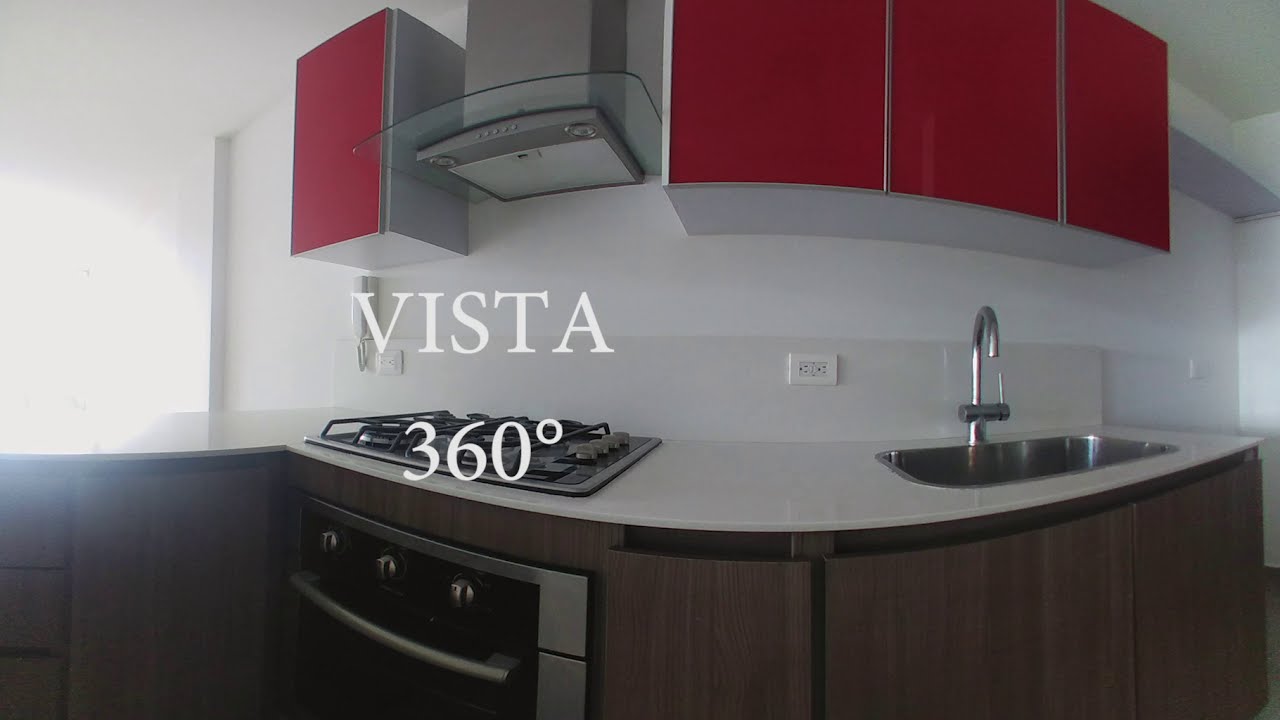This photograph captures the interior of a contemporary kitchen, marked by a central white countertop. On the left side of the counter rests a cooktop with a black oven underneath, featuring silver knobs and illuminated by a stove light above. Directly above this cooking area is a grey chimney. To the right of the counter, a stainless steel, silver sink is positioned. Below the white counter, dark brown wooden cabinets provide storage.

The kitchen features all-white walls and ceiling, contributing to a clean and minimalist atmosphere. Mounted on the wall, there are a few electrical sockets, and above the countertop, four red cabinet sections with a slight white border stand out. Natural light filters in from the left side of the image, casting a gentle illumination across the countertop and walls.

The image appears slightly curved, likely due to a filter applied to create a panoramic effect. Superimposed on top of the image, in white graphical text, are the words "Vista 360 degree." This text is centrally placed over the countertop and stove area, emphasizing the comprehensive view of the kitchen.